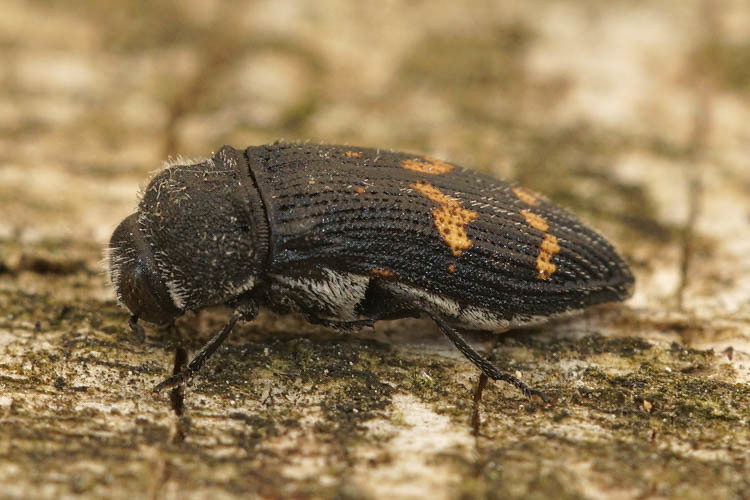This detailed photograph captures a striking insect, likely a beetle, perched on a piece of wood that is brown with white speckles. The insect itself is a large, dark-colored creature with prominent features. Its body, predominantly black or dark brown, is adorned with distinctive orange or yellowish spots and lines, appearing almost as if bleach had splashed onto its back. The beetle has short white hairs scattered over its body, giving it a somewhat furry appearance. It boasts large, round eyes and four visible legs, with others perhaps blending into the wood's texture. The background is tastefully blurred, featuring hues of green and brown, suggesting an outdoor setting that complements the colors of both the insect and the wood. The overall image is sharply focused on the insect and the wood, offering a detailed glimpse into the intricate features of this fascinating beetle.